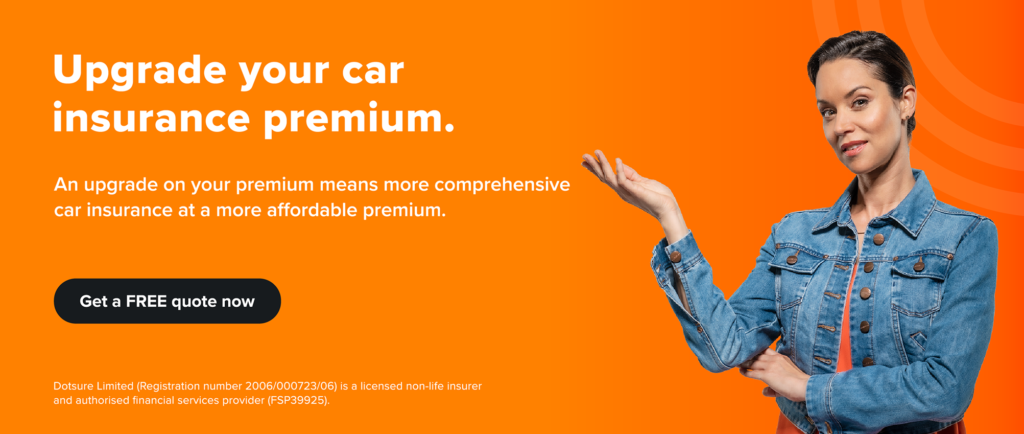An orange-themed advertising banner features a gradient background that transitions from a lighter shade on the left to a darker shade on the right. In the upper right corner, three curved stripes in a lighter orange shade add a visual accent. Standing in front is a young woman with short brown hair, wearing an orange t-shirt and a jean jacket. She poses with her left arm across her body, supporting her right elbow, while her right hand is outstretched. She gazes at the camera with a slight smile. 

On the left side of the banner, white text reads: "Upgrade your car insurance premium. An upgrade on your premium means more comprehensive car insurance at a more affordable premium. Dotsure Limited, registration number 260072306, is a licensed non-life insurer and authorized financial services provider." 

A black button with white text at the bottom invites viewers to "Get a Free Quote Now."